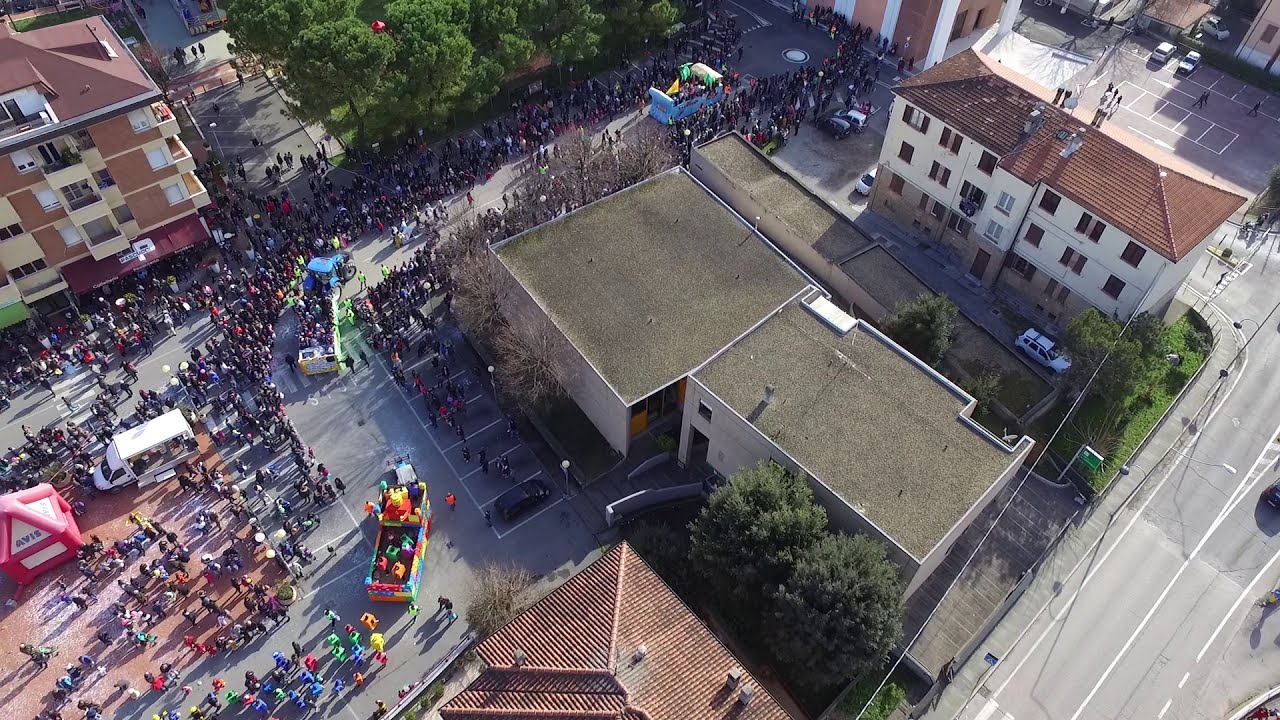This is a vibrant, detailed aerial photograph of a city parade taken on a clear, sunny day. The rectangular image captures an expansive view from high above, possibly from the top of a tall building, offering a broad perspective that encompasses various cityscape elements. The parade winds through several streets, which wrap around a collection of diverse buildings, some with flat roofs and others donning traditional terracotta styles. Along these streets, throngs of people form lively crowds, cheering and watching the procession below. The parade features three colorful floats, each adorned with bright hues like yellow, blue, red, and orange. One float is particularly bustling, with people riding on it and others marching behind in vivid attire. An eye-catching red inflatable awning, emblazoned with "Avis," punctuates the scene on the right-hand side. Adding to the urban texture, a few parking structures sit in front of the buildings, while some spectators even gather on the rooftops for a better view. The festive energy of the parade juxtaposed against the orderly cityscape makes for a richly detailed and dynamic photograph.